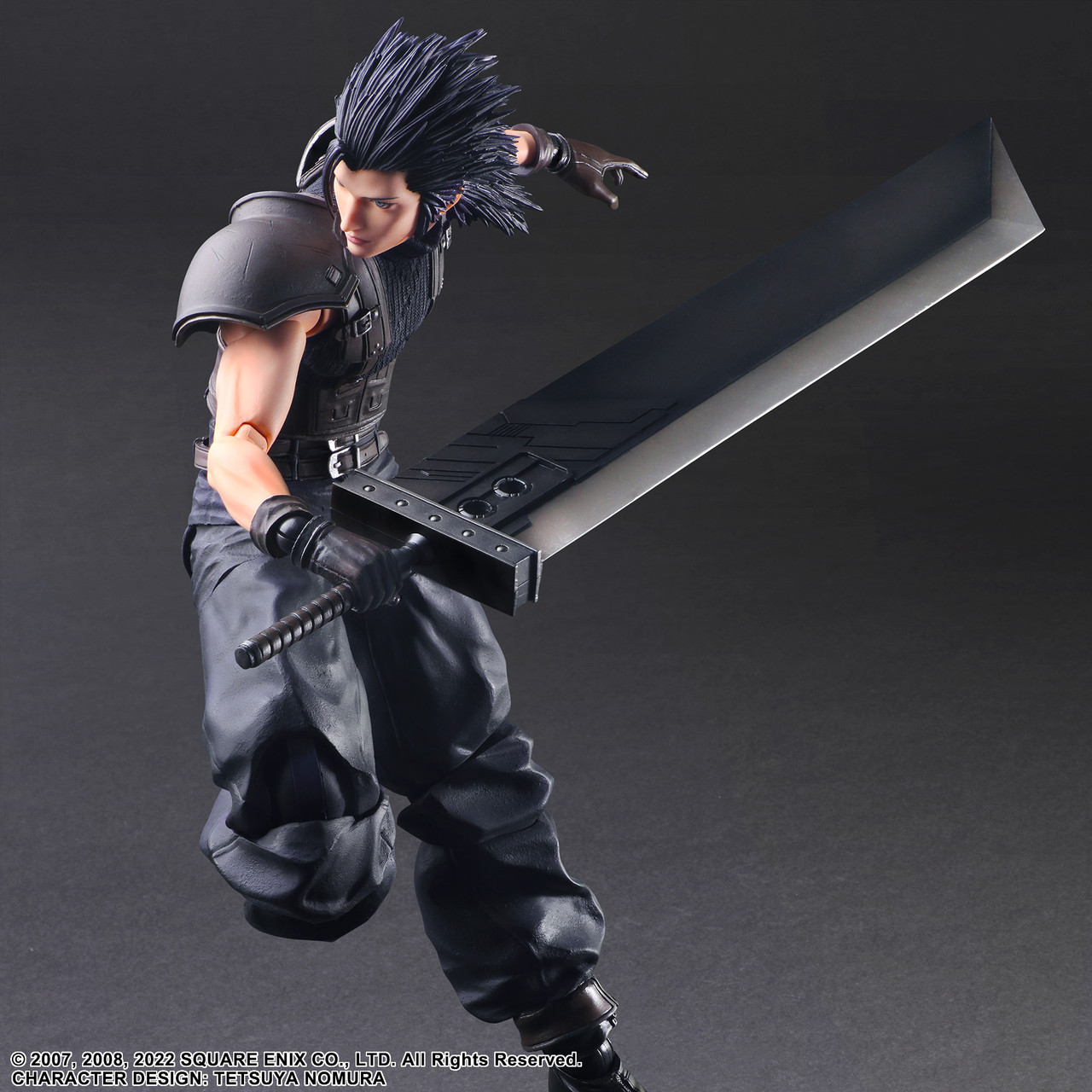The image depicts an anime figure of a video game character, reminiscent of Cloud from Final Fantasy VII, known for his iconic massive sword. The figure is portrayed in a dynamic action pose, standing on his left leg with his right leg bent and raised behind him, as if poised to strike. The character brandishes a massive blade in his right hand, extended outward, while his left arm is drawn back. His long, slicked-back, dark hair adds to his striking appearance.

He is dressed in an ensemble of baggy black pants, black boots, a sleeveless black shirt, and features black gloves. A distinct black shoulder pad adds a touch of armor to his look. The backdrop of the image transitions from dark gray at the top to a lighter gray at the bottom. The bottom left corner of the image features text that reads: "2007-2008-2022 Square Enix Company Limited. All Rights Reserved. Character Design: Tetsuya Nomura."